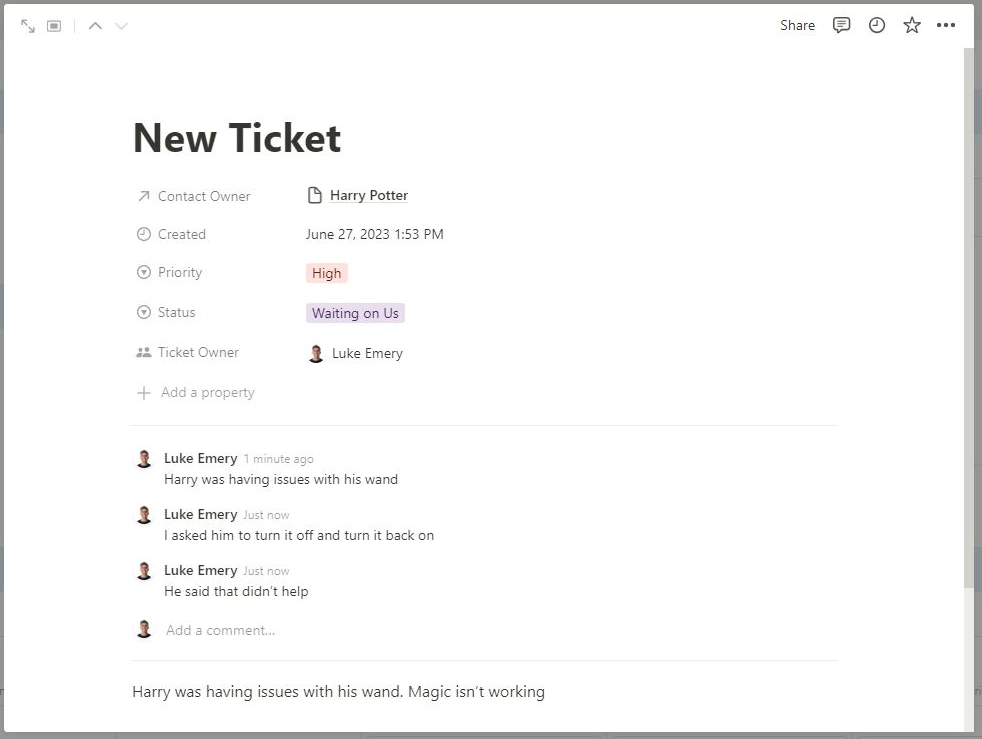The screen capture showcases a detailed interface on a white background, populated with various colored fonts and a plethora of icons. At the very top are two arrow icons adjacent to a square-within-a-square icon, followed by scroll buttons, a 'Share' option, and icons depicting a text bubble, clock, star, and three gray circles.

The central portion prominently displays a new ticket interface:
- The header reads "New Ticket"
- The point of contact is listed as "Owner: Harry Potter" followed by an arrow icon.
- The ticket creation details include a clock icon and the timestamp: "June 27, 2023, at 1:53 p.m."
- The priority status is denoted by an arrow next to the word "High" in pink.
- The ticket's current status, indicated in purple text, reads "Waiting on Us"
- Below, "Ticket Owner" is accompanied by small people icons. The owner's name, "Luke Emery," is shown along with a small, round photo of a man wearing a blue shirt and a plus sign.

In the comments section beneath this:
- "Luke Emery, one minute ago: Harry was having issues with his wand."
- "Just now: I asked him to turn it off and turn it back on."
- "Luke Emery, just now: He did that. It didn’t help."

Each comment is paired with Luke Emery's picture, and an option to "Add a comment" is available below this thread.

At the bottom, a repetitive note states: "Harry was having issues with his wand. Magic isn't working."

Along the right side of this interface, there is a visible gray scroll bar.